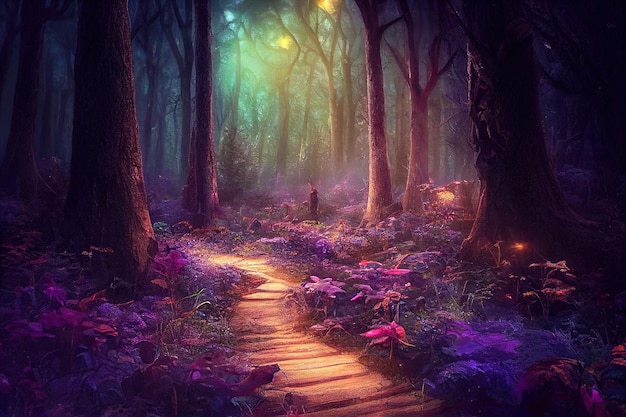This detailed digital painting depicts a fantastical, enchanted forest brimming with an otherworldly atmosphere. Central to the scene is a meandering pathway composed of light brown wooden planks lined with vibrant purple flowers and grasses. The forest is populated with leafless trees featuring dark purple trunks, while glowing yellow insects add a surreal luminescence to the air. The dense canopy allows light green sky and spots of blue to peek through, illuminating the center pathway in a mystical glow. The fringes of the scene are enveloped in shadowy darkness, punctuated by two eerie orange spots on either side. Although subtle and somewhat blurred, the silhouette of a figure can be discerned standing along the pathway, lending an enigmatic focal point to the artwork's enchanted ambiance.